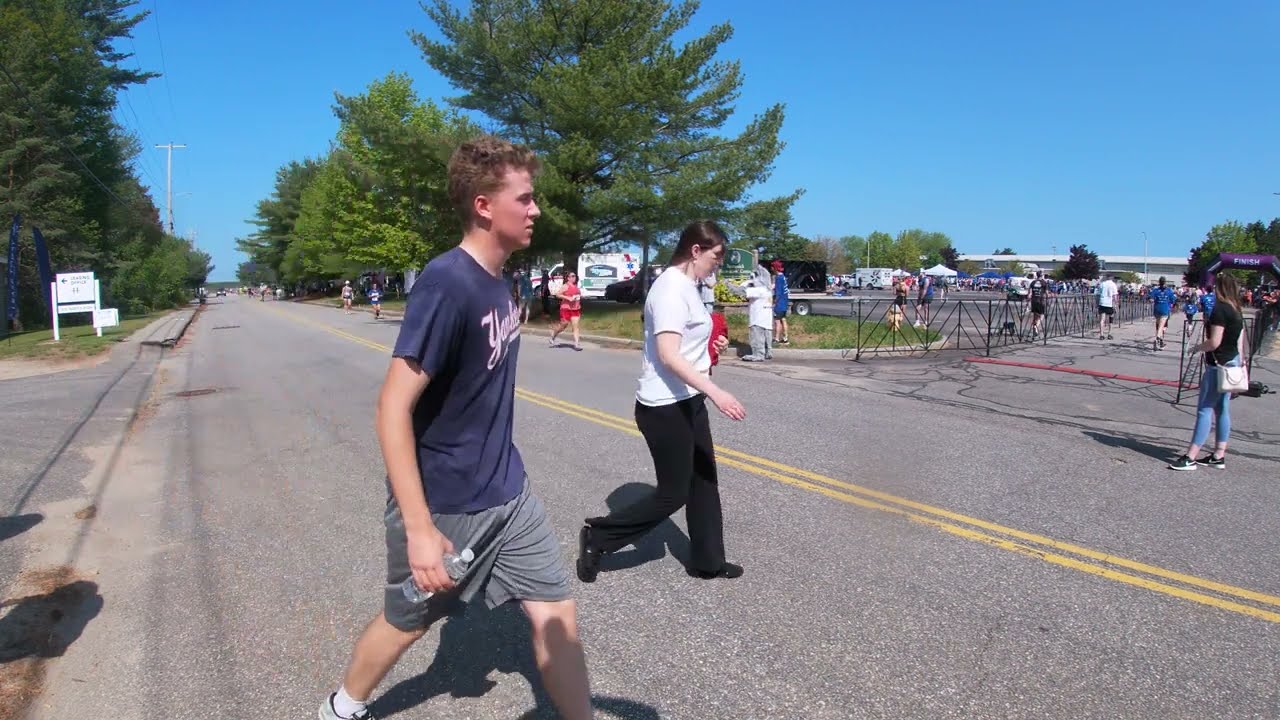The photograph captures a dynamic street scene on a bright, cloudless day. The street, delineated by a faded double yellow line, extends diagonally from the lower right-hand corner to the upper left, cutting through a lush landscape with towering, vibrant green trees on either side. In the foreground, close to the camera, a young man with short, light brown curly hair, drenched in sweat, walks across the street. He’s clad in a navy blue shirt emblazoned with "Yankees" and gray shorts, carrying a water bottle in his right hand. To his left and slightly ahead, a young woman with dark brown hair tied back in a ponytail walks alongside him. She wears a white short-sleeved polo shirt, black slacks, and black shoes, carrying a small red object in her left arm. In the background, more people can be seen; some are running towards the foreground, likely participants in a race, while others observe from the roadside. The deep, brilliant blue sky without a single cloud emphasizes the clarity of the scene, making the green foliage and street details stand out vividly.